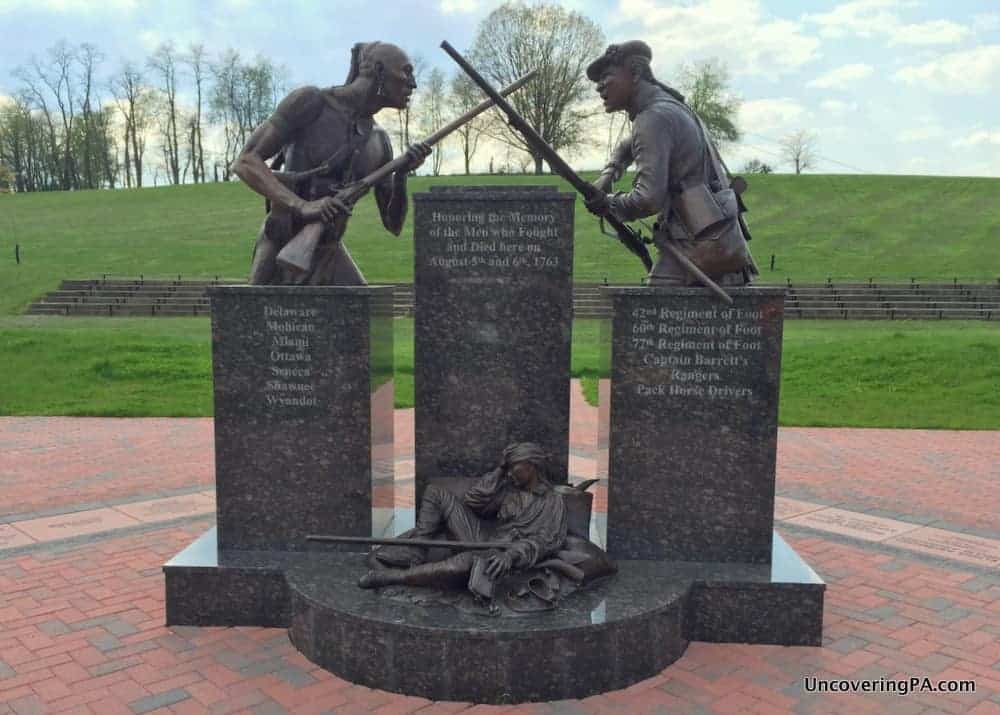In an outdoor setting under a blue sky with white clouds, this meticulously detailed memorial sculpture captures a poignant moment from history. The centerpiece is composed of three granite pillars atop a red brick platform, intricately crafted to honor the memory of men who fought and died in a battle on August 5th and 6th, 1763. Surrounding the platform is a concrete block border, set amidst a lush green garden with trees and a gentle grass-covered hill in the background.

On the left pillar stands a shirtless Native American man, depicted with his hair pulled back into a ponytail and an earring, symbolically holding a rifle. The center, taller pillar serves as the main focal point with engraved tributes, its precise carvings capturing the gravity of the memorial. On the right pillar is a soldier from the 42nd Regiment, portrayed in a historic 1700s military outfit complete with a braid down his back and a single-shot musket in hand, facing the Native American figure in a significant stance.

At the base of these pillars, a fallen soldier lies with his musket, evoking a sense of grief and sacrifice. The entire memorial rests on a reddish and black brick plaza, adding to the solemn ambiance. Details such as names and regiment information are engraved on the pillars, though some inscriptions are blurred and difficult to decipher. In the corner of this evocative scene, the black font marks uncoveringpa.com, hinting at further historical insights about this commemorative site.